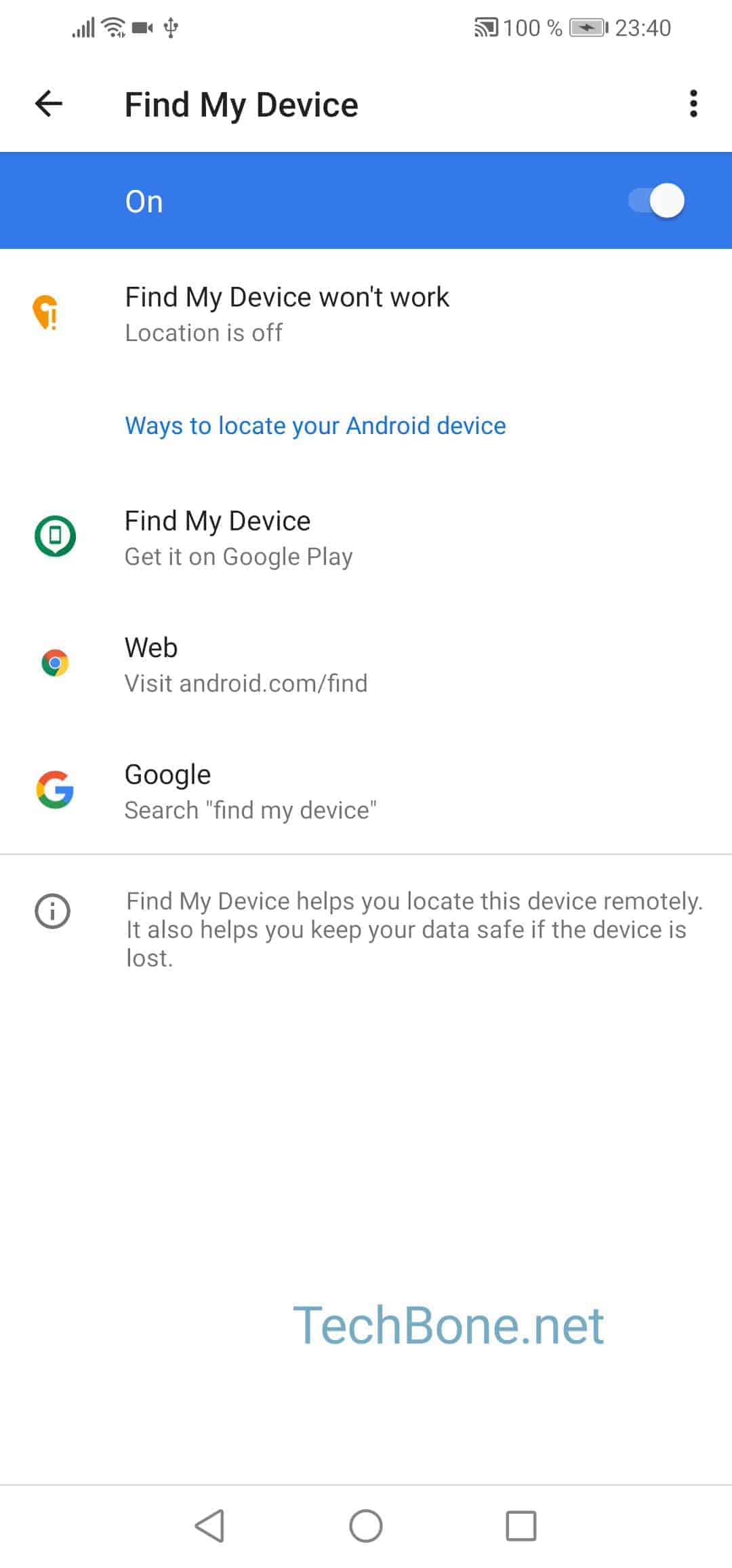This image showcases the homepage of the "Find My Device" feature on an Android smartphone. At the top of the screen, the smartphone's status bar displays several icons and indicators. 

On the top right, there is an icon for screencasting, a fully charged battery icon that is currently charging, and the time displayed as 23:40. On the top left, there is a collection of four icons: Wi-Fi, network connectivity, a video icon, and a USB connection icon which is grey.

The main screen is open to the "Find My Device" application, set against a blue background. The header prominently displays "Find My Device" with its status indicated as "On." To the right of this text is a switch toggle, which is currently switched on.

Below the header, there are several options and informational sections. 
1. The first section alerts the user with an orange exclamation mark and a location pin icon, stating "Find My Device won't work" if location services are turned off. This warning is followed by a blue text link reading, "Where to locate your Android device," with the rest of the text in black.
2. The second option provides a quick guide to using "Find My Device" through various methods:
    - "Quickly play a sound," accompanied by a green and white icon.
    - "Visit android.com/find on the web," with a Chrome icon indicating this option.
    - "Quickly search 'Find My Device'," symbolized by a multi-colored glyph in blue, green, yellow, and red.

At the bottom of the screen, it explains the function of "Find My Device," emphasizing its utility in locating the device remotely and securing data if the device is lost. This is followed by a reference to the website "techbone.net," highlighted in blue text.

This detailed caption comprehensively describes the key elements and functionalities displayed in the smartphone screenshot.